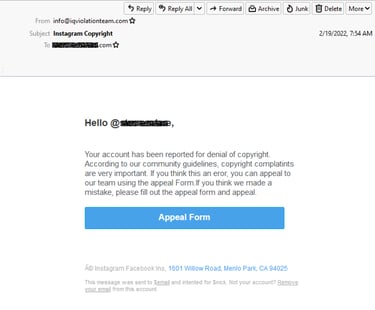This image shows a screenshot of an email opened in an email application. At the very top of the interface, a header section displays information fields for "From," "Subject," and "To" on the left side. Next to these fields are several buttons: "Reply," "Reply All," "Forward," "Archive," "Junk," "Delete," and "More," each aligned to the right corner.

The "From" field indicates that the email is from "info.iqviclationteam.com," beside which a prominent black star is visible. The "Subject" field reads "Instagram copyright." The "To" field contains redacted information masked by "blackmarker.com." On the far right side of the header, a timestamp indicates the email was received on February 19, 2022, at 7:54 AM.

The body of the email message starts with "Hello," followed by a redacted name. The email informs the recipient that their account has been reported for a copyright violation. It emphasizes the importance of copyright complaints as per Instagram's community guidelines and provides information on how to appeal the decision if the recipient believes it was made in error. A blue button labeled "Appeal Form" is prominently positioned towards the bottom of the email body for this purpose.

The email also includes a small-print footer with the address "Instagram, Facebook, 1601 Willow Road, Menlo Park, California, 94025." There is additional fine print that begins with "This message was sent to," but the rest of this text, along with the sentence "Not your account," is blurry and hard to read.